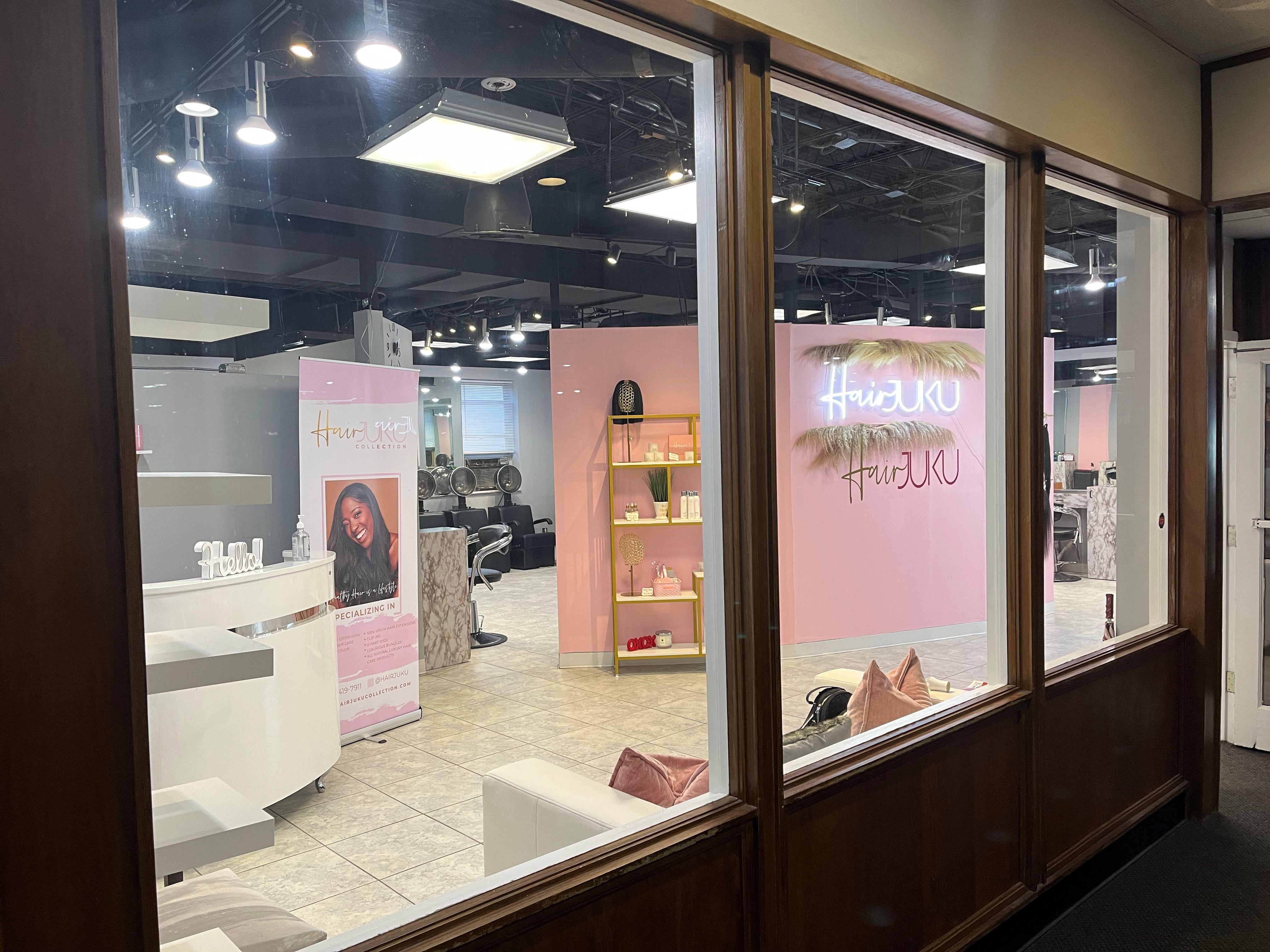The photograph captures the well-lit storefront of a beauty salon, contrasting the dark exterior environment. The facade comprises three large, brown-trimmed window panes, with a white ceiling above them. Peering through the glass reveals a stylish interior featuring a gray and white tiled floor, pink display features, and a welcoming white countertop adorned with a "hello" sign. The salon's name, "Hair Juku," is prominently displayed in both white and red text amidst an inviting decor that includes palm tree accents. Inside, there is a gold shelf brimming with beauty products and a cozy white loveseat positioned against the window. Additionally, a pink wall serves as a backdrop for a shelf filled with various products, while a large poster depicts a woman with long black hair, enjoying a manicure. The serene and inviting atmosphere is accentuated by the presence of hair dryers and comfy chairs tucked away in the back of the salon, ensuring a luxurious experience for its patrons.